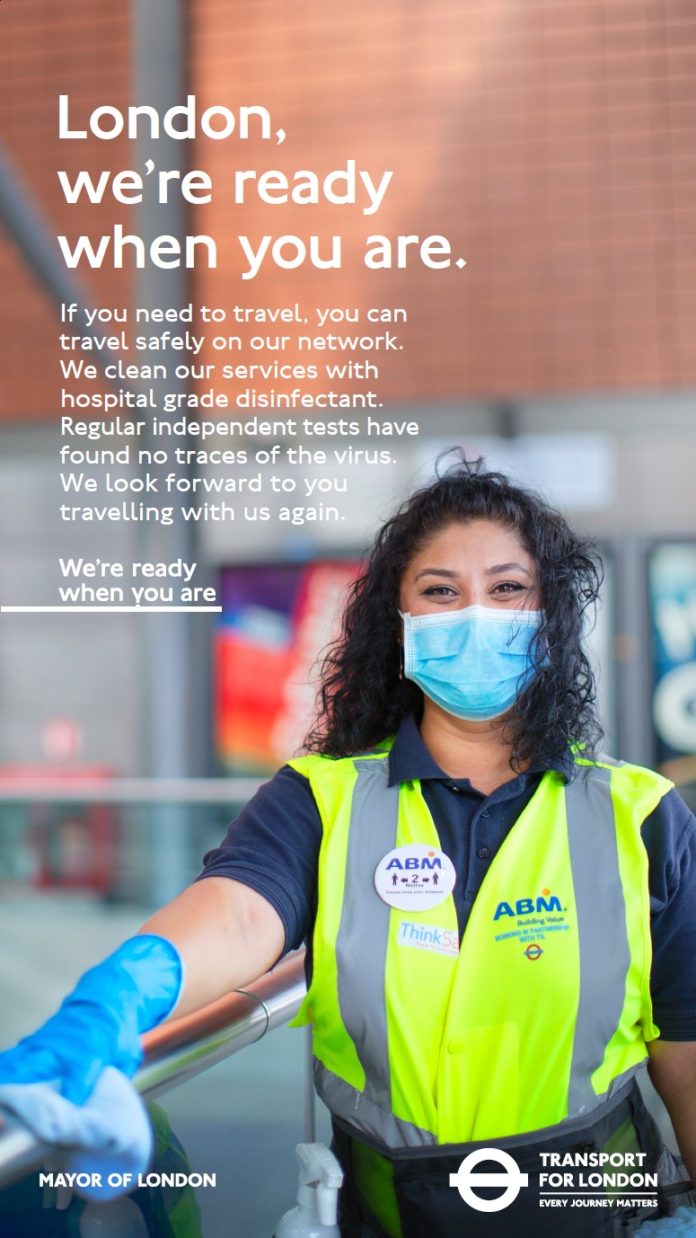This advertisement features a photograph of a young woman with long, curly, dark hair cascading past her shoulders, looking directly at the camera. Despite wearing a blue surgical mask, her smiling eyes convey a welcoming expression. She is dressed in a neon yellow reflective vest emblazoned with a circular badge on the left side bearing the initials "ABM" and text on the right side that reads "ABM Building Value." The woman is reaching out with her right hand, which is protected by a blue latex glove, and diligently wiping down a handrail with a blue cloth.

The advertisement's text pronounces: "London, we're ready when you are. If you need to travel, you can travel safely on our network. We clean our services with hospital-grade disinfectant. Regular independent tests have found no traces of the virus. We look forward to you traveling with us again. We're ready when you are. Mayor of London, Transport for London, Every Journey Matters."

The image is in a portrait orientation, devoid of animals, plants, flowers, trees, automobiles, or airplanes, focusing solely on the commitment to cleanliness and safety within London's transport network.